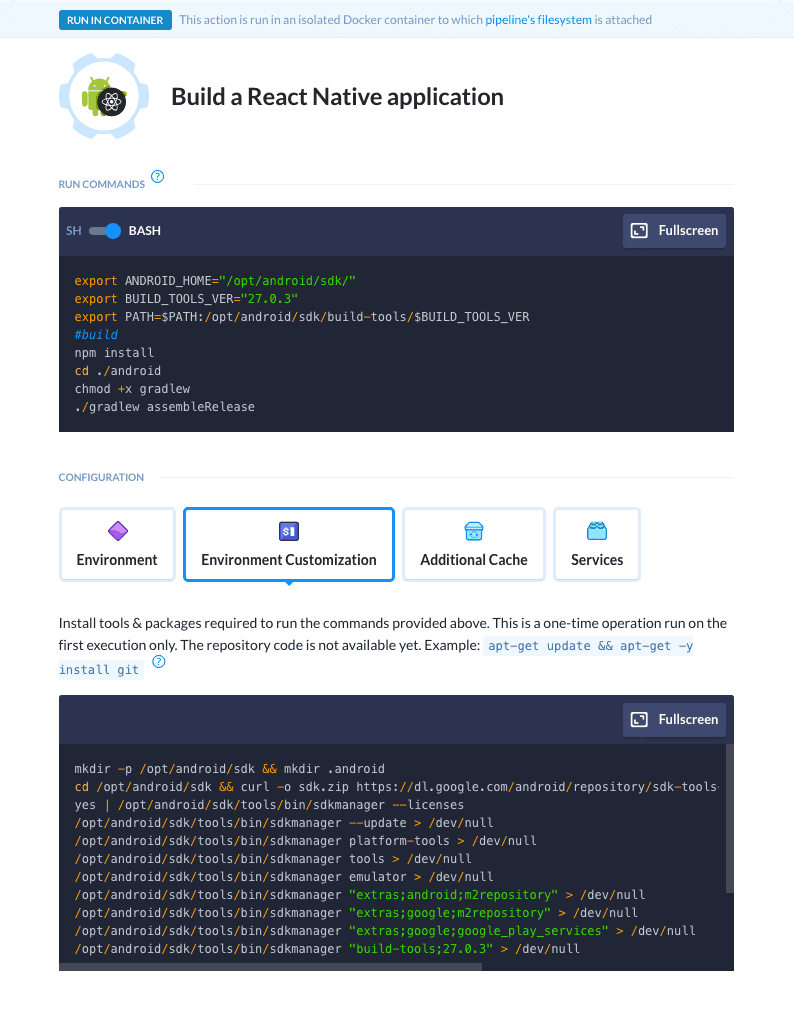### Detailed Caption for Technical Image:

The screenshot displays a complex coding environment, highlighted by its intricate technical data. The interface prominently features the heading "Run in Container" at the top, indicating that the action is executing within an isolated Docker container, with the pipeline's file system attached. In the top-left corner, an advanced logo combines a gear avatar, a robot, and a nuclear symbol, enhancing the high-tech aesthetic.

Just below, the caption "Build a React Native Application" is visible next to a question mark, suggesting an interactive or customizable build process. The background is a deep navy blue, adding to the sophisticated look of the environment.

The code execution section is highlighted with "SH Bash," showing that the shell is set to Bash. This area includes buttons for various functions, including environment customization, additional cache, and services, as well as the option to make the view full screen, located in the upper right corner.

Commands for this technical interface include "export," "build," "NPM," "cd," "chmod," and others. Specific installations such as "apt-get update" and "apt-get -y install git" are mentioned, indicating steps for setting up the required tools and packages for the environment.

At the center of the image, buttons provide various customization options. It's noted that some operations, like installing necessary tools and packages, are one-time tasks, performed during the first execution.

Overall, this screenshot is clearly tailored for a technical audience, providing detailed and essential coding and command execution options for building a React Native application within Docker.